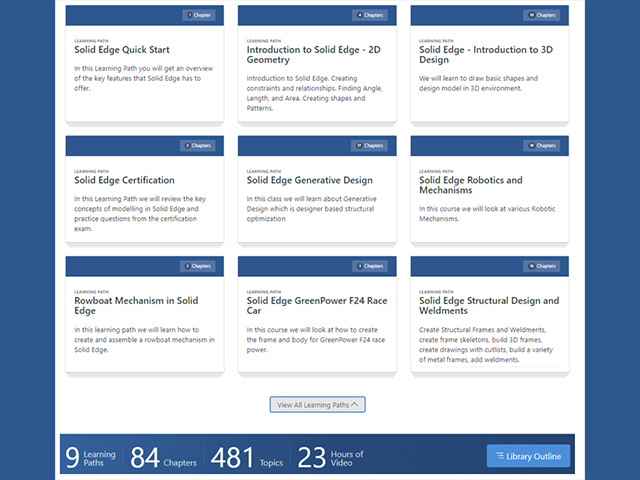The web page features a dark blue background with multiple instances displayed in various squares on the left-hand side, all with dark blue bezels. Each square has a heading labeled "Chapters" with a dark blue circle next to it.

1. The first square is titled "Learning Path" with the bold text "Solid Edge Quick Start," followed by a description: "In this learning path, you will get an overview of the key features that Solid Edge has to offer."
2. The next one also begins with "Learning Path" and is titled "Introduction to Solid Edge – 2D Geometry," detailing various topics such as creating constraints and relationships, as well as finding angles, lengths, and areas, and creating shapes and patterns.
3. This is followed by "Solid Edge – Introduction to 3D Design," which talks about learning to draw basic shapes and design models in a 3D environment.
4. Another entry is "Solid Edge Certification," explaining: "In this learning path, we will review the key concepts of modeling in Solid Edge and practice questions from the certification exam."
5. "Solid Edge Generative Design" follows, explaining: "In this class, we will learn about generative design, which is designer-based structural optimization."
6. Continuing, "Solid Edge Robotics and Mechanisms" mentions: "In this course, we will look at various robotic mechanisms."
7. "Rowboat Mechanical Mechanism in Solid Edge" describes: "In this learning path, we will learn how to create and assemble a rowboat mechanism in Solid Edge."
8. "Solid Edge Green Power F24 Race Car" explains: "In this course, we will look at how to create the frame and body of a Green Power F24 racecar."
9. The last one on the left side, titled "Solid Edge Structural Design and Weldments," covers topics like creating structural frames and weldments, building 3D frames, and creating detailed drawings with a cut list, among other things.

On the right-hand side, there is a dark gray clickable rectangle bordered in dark blue labeled "View All Learning Paths" with an upward arrow icon.

There is also a rectangle in mid-blue with dark hash lines cascading down, which reads "Library Online" in white text. Another section presents statistics in bold white text: "9 Learning Paths," "84 Chapters," "481 Topics," and "23 Hours of Video."

The details convey a comprehensive overview of the various learning paths and courses available on the web page, focusing on different aspects and functionalities of Solid Edge.